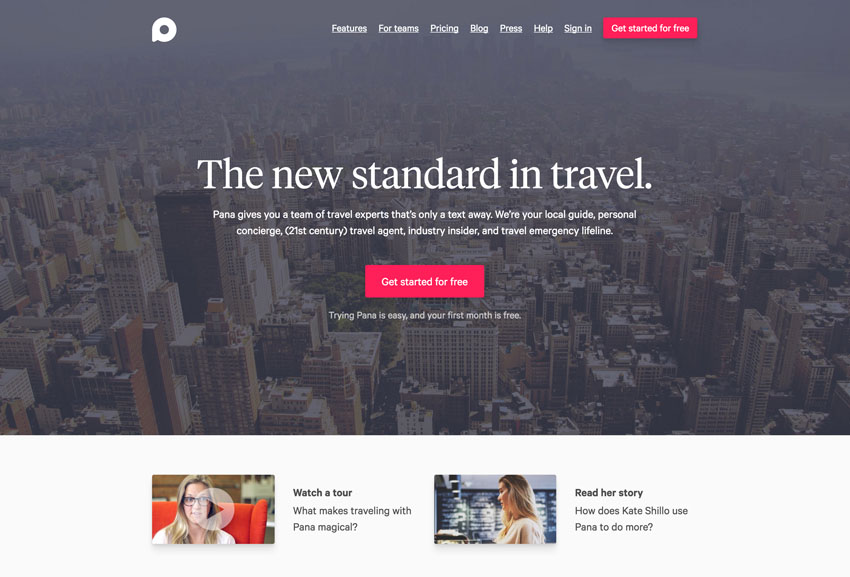**Caption:**

"Explore the future of travel with Pana, the new standard in personalized travel services. This advertisement showcases a bustling metropolitan city with towering skyscrapers, shaded in a dark overcast that highlights the cityscape's grandeur. Pana offers a 21st-century travel experience with a team of travel experts, local guides, personal concierges, and an emergency lifeline - all just a text away. 

The top navigation bar features options for Teams, Pricing, Blog, Press Releases, Help, and Sign In, inviting users to create an account and get started for free. A prominent red button at the bottom encourages visitors to take advantage of a free month trial. Also at the bottom, you can watch a video tutorial to see what makes traveling with Pana magical, along with an inspiring testimonial from Kate Shiloh on how Pana enhances her travel experience. Two women, Caucasian with long blonde hair, are also shown — one facing the camera while sitting in an orange chair, the other in an office setting, adding a personal touch to the ad."